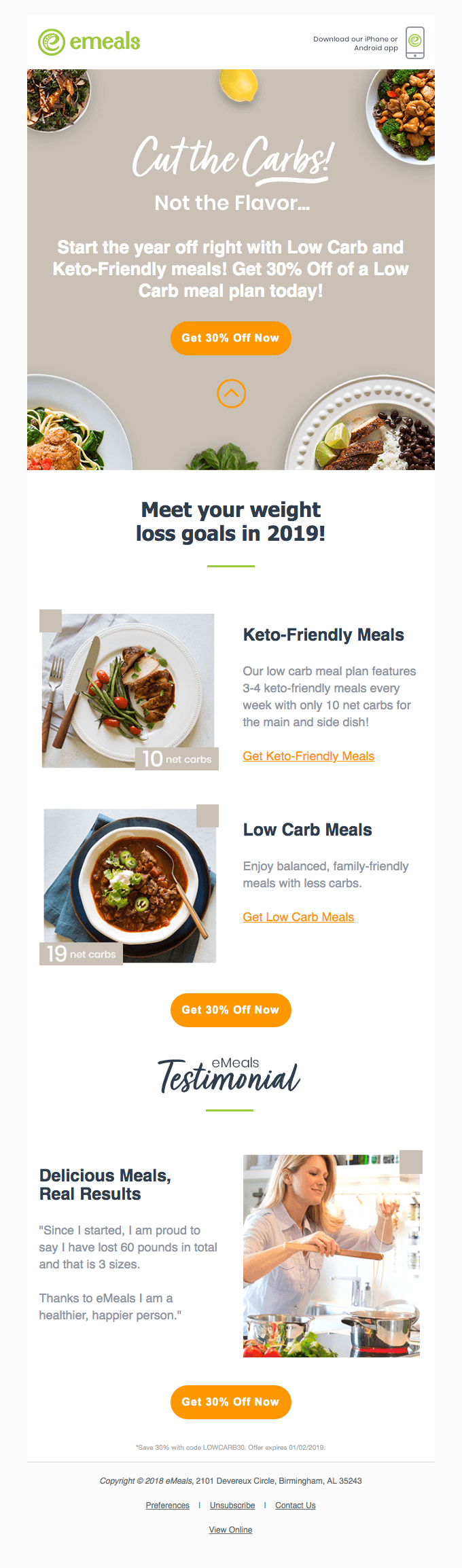The screenshot depicts a webpage from the healthy eating and lifestyle website "E-Meals," as evident from the logo in the top left-hand corner, which is displayed in light green font. Dominating the top of the page is a promotional banner with the caption: "Cut the carbs, not the flavor. Start the year off right with low-carb and keto-friendly meals. Get 30% off of a low-carb meal plan today." Just below this caption, there's an elongated, orange, oval-shaped button with the text "Get 30% off now."

Throughout the page, there are various appealing images of different healthy dishes, emphasizing the website's focus on nutritious meals. Featured in the bottom right-hand corner is a photograph of a woman cooking in a kitchen, likely preparing her own meal. The promotional button "Get 30% off now" is repetitively displayed three times on the page, encouraging visitors to take advantage of the discount.

The webpage has a clean and simple design with a white background and black text. The overall layout suggests an inviting and accessible resource for individuals interested in improving their diet and lifestyle through low-carb options.